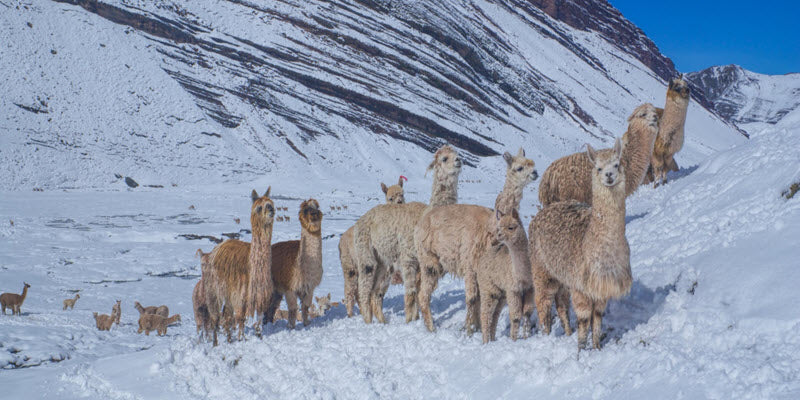The photograph captures a picturesque scene of a pack of llamas on a snow-covered mountainside under a clear, blue sky. The setting appears to be a remote and deserted mountain area, with steep slopes showcasing horizontal striations of stone intermingled with pure white snow. There are approximately 10 to 15 llamas, predominantly light brown or tan in color with some variations of darker brown, all adorned with fluffy coats that suggest warmth despite the frigid surroundings. Most of the llamas, some with distinctive white faces, are gathered closely to the camera, keenly observing the photographer, while others can be seen scattered further into the snowy expanse. Their presence provides a stark contrast against the pristine snow, emphasizing the serene and untouched beauty of the mountainous wilderness.